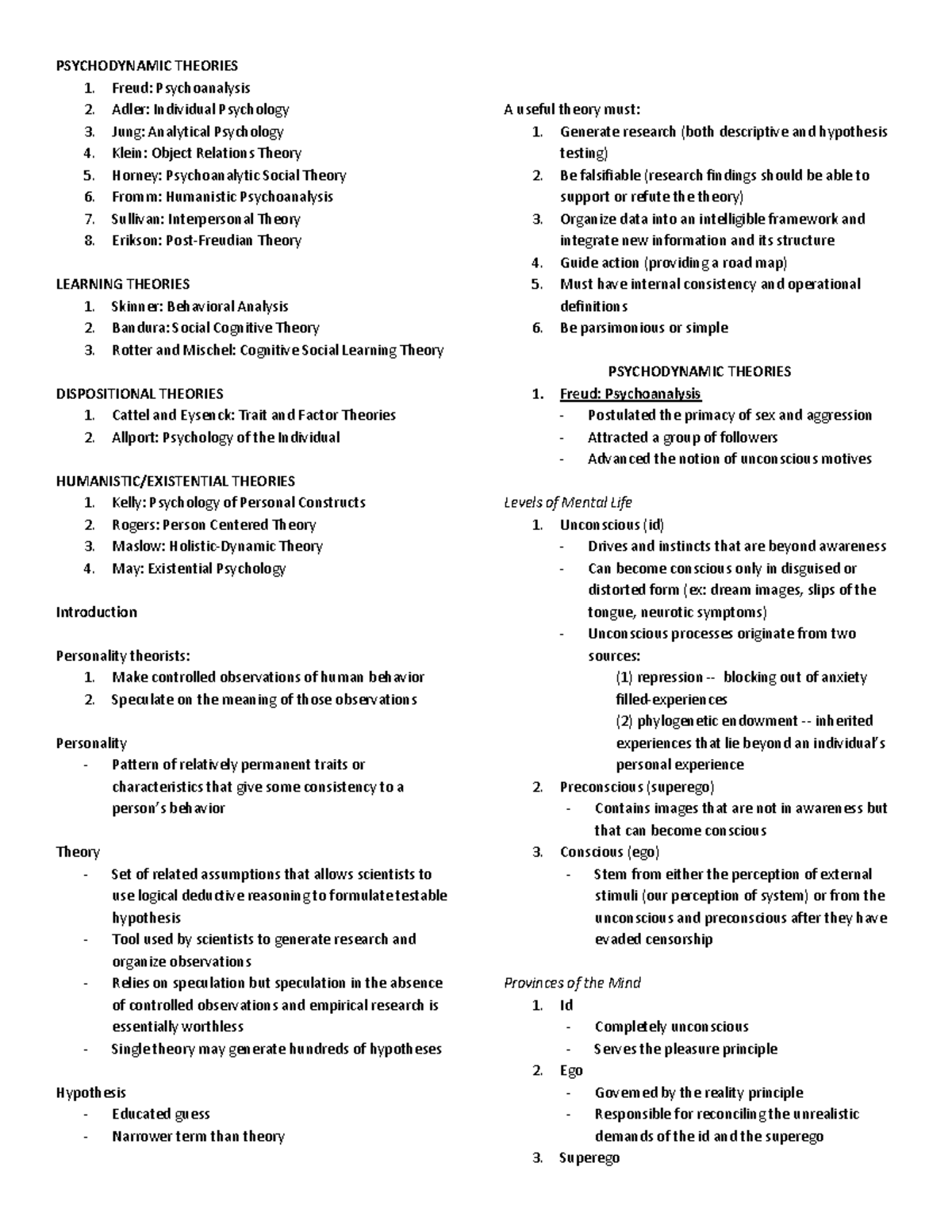**Image Caption: Detailed Table of Psychodynamic Theories and Theories of Personality**

The image displays a comprehensive table categorizing various psychological theories against a white backdrop, with all text in black. 

**Psychodynamic Theories**:
1. Freud - Psychoanalysis
   - Postulated the primacy of sex and aggression.
   - Attracted a group of followers.
   - Advanced the notion of unconscious motives.
   - Levels of mental life:
     - **Unconscious (ID)**: Drives and instincts beyond awareness, can become conscious only in disguised/distorted form (e.g., dream images, slips of the tongue, neurotic symptoms). Originates from two sources: repression (blocking anxiety-filled experiences) and phylogenetic endowment (inherited experiences beyond personal experience).
     - **Preconscious (Superego)**: Contains images not in awareness but can become conscious.
     - **Conscious (Ego)**: Stems from the perception of external stimuli (perceptual system) or from the unconscious and preconscious after evading censorship.
   - Provinces of the mind:
     - **ID**: Completely unconscious, serves the pleasure principle.
     - **Ego**: Governed by the reality principle, reconciles the unrealistic demands of the ID and superego.
     - **Superego**.
   
2. Adler - Individual Psychology.
   
3. Jung - Analytical Psychology.
   
4. Klein - Object Relations Theories.
   
5. Horney - Psychoanalytic Social Theory.
   
6. Fromm - Humanistic Psychoanalysis.
   
7. Sullivan - Interpersonal Theory.
   
8. Erikson - Post-Freudian Theory.

**Learning Theories**:
1. Skinner - Behavioral Analysis.
   
2. Bandura - Social Cognitive Theory.
   
3. Rotter & Mischel - Cognitive Social Learning Theory.

**Dispositional Theories**:
1. Cattell & Eysenck - Trait and Factor Theories.
   
2. Allport - Psychology of the Individual.

**Humanistic/Existential Theories**:
1. Kelly - Psychology of Personal Constructs.
   
2. Rogers - Person-Centered Theory.
   
3. Maslow - Holistic Dynamic Theory.
   
4. May - Existential Psychology.

**Introduction to Personality Theorists**:
1. Make controlled observations of human behavior.
2. Speculate on the meaning of these observations.

**Definitions**:
- **Personality**: Pattern of relatively permanent traits or characteristics that give some consistency to a person's behavior.
- **Theory**: Set of related assumptions that allow scientists to use logical deductive reasoning to formulate testable hypotheses. A tool used by scientists to generate research and organize observations. Relies on speculation, but speculation in the absence of controlled observations and empirical research is essentially worthless. A single theory may generate hundreds of hypotheses.
- **Hypothesis**: An educated guess, a narrower term than theory.

**Criteria for a Useful Theory**:
1. Generate research (both descriptive and hypotheses of testing).
2. Be falsifiable (research findings should support or refute the theory).
3. Organize data into an intelligible framework and integrate new information.
4. Guide action (providing a roadmap).
5. Have internal consistency and operational definitions.
6. Be parsimonious or simple.

This meticulously organized table serves as an extensive reference for students and scholars delving into the intricate world of psychological theories.